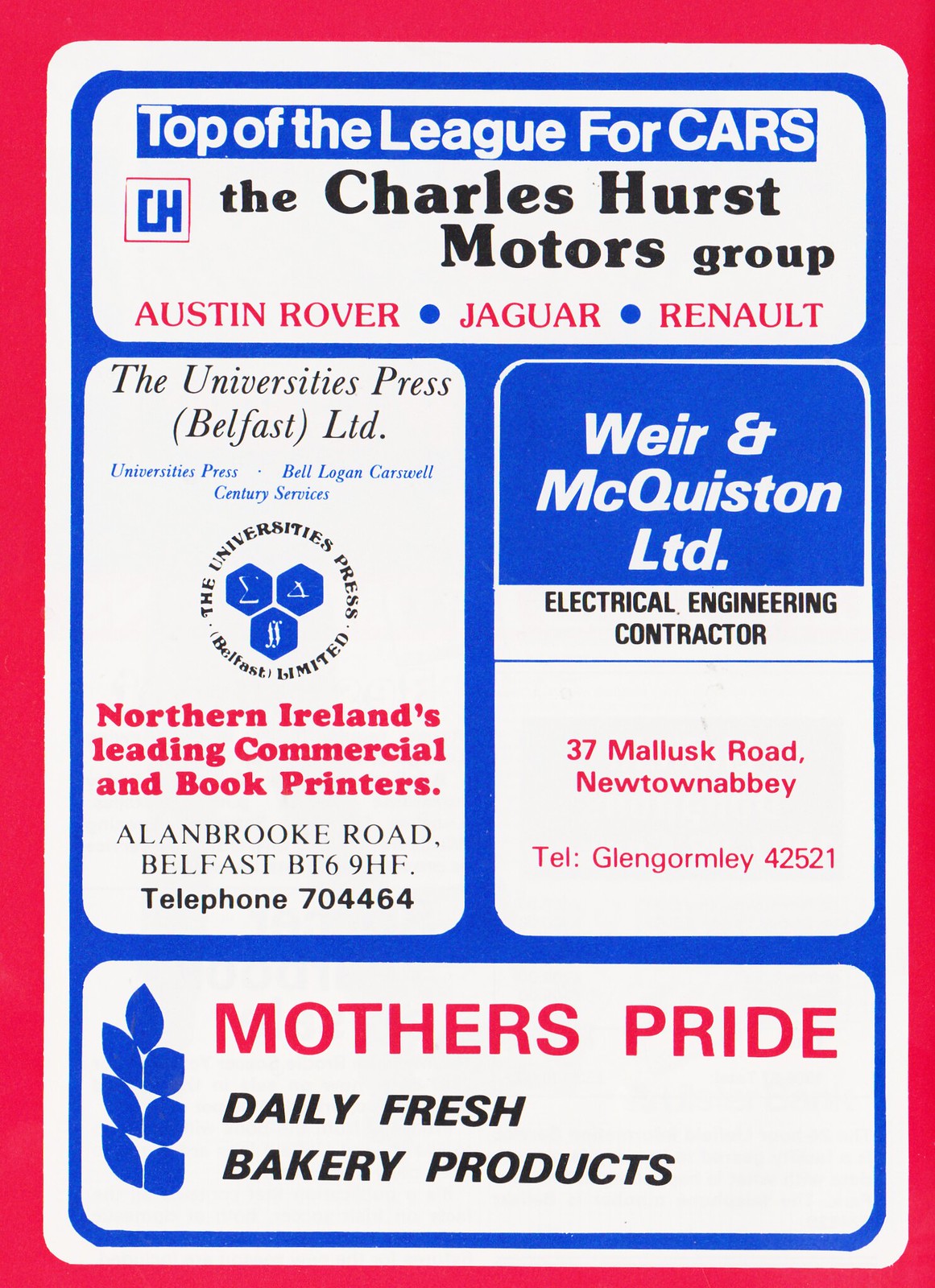The image is a detailed advertisement featuring multiple sections, each with distinct content. The advert has a prominent red border encasing a white background, further framed by a bright blue inner border. At the top, in a blue-highlighted rectangle with white text, the banner reads "Top of the League for Cars." Below this, a red circle with "CH" introduces the Charles Hurst Motor Group, alongside the names "Austin Rover, Jaguar, Renault" in red text.

The middle section comprises two adjacent rectangular boxes. The left box is tagged as "University Press Belfast LTD" with the claim "Northern Ireland's Leading Commercial and Book Printers" written in red. It also includes the address "Allenbrook Road, Belfast BT6 9HF" and the telephone number "704464" in black.

To the right, the second middle box, highlighted in blue with white text, features "Weir & McQuiston LTD," a company described as "Electrical Engineering Contractor." It lists the address "37 Malusk Road, Newton Abbey" and telephone number "Glen Gormley 42521" in black text.

At the bottom of the advertisement, a wide horizontal rectangle showcases a blue outline of wheat and the brand name "Mother's Pride" in red. Below this, it advertises "Daily Fresh Bakery Products" in black text.